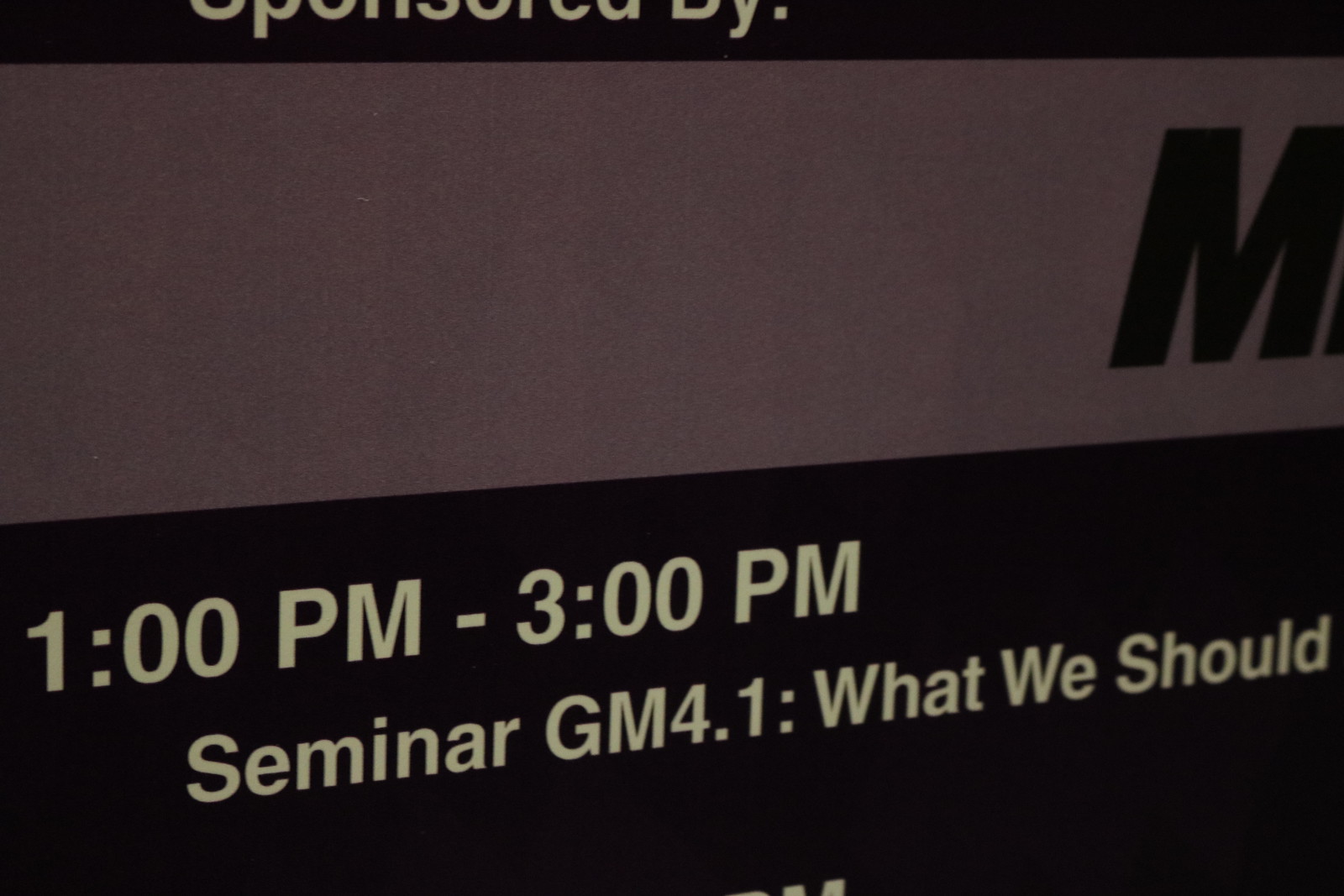The image depicts a sign or poster, possibly on a wall or a presentation slide, with a predominantly black background. At the very top edge, there's partially visible text in a brownish-cream color against the black background, which appears to say "sponsored by." Directly beneath this is a horizontal gray banner extending across the width of the image, where the right edge reveals an "M" in black. The lower half of the image contains another black section featuring green and white text. The green text indicates a time range: "1:00 PM - 3:00 PM." Below this, in white text, it reads: "seminar gm 4.1: what we should" (the rest of the text is cut off). The image is taken at a slight angle, emphasizing the colors black, white, gray, and green.